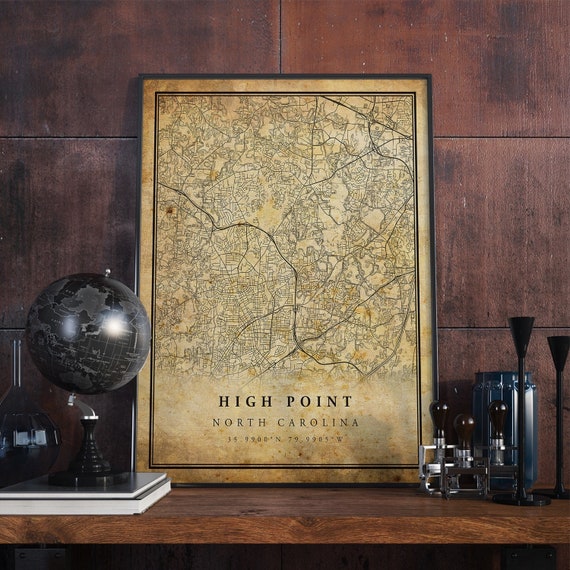A color photograph captures an intriguing arrangement of objects on a dark wooden shelf, positioned against a distressed, reddish-brown wall made up of rectangular panels. On the far left, partially out of frame, sits a small glass vase with a slender neck. Adjacent to it is a small black globe with gray countries, perched atop two books—a thick one and a thin one. The centerpiece of the collection is a vintage-looking framed map with a black frame. The yellowing paper of the map displays the streets of High Point, North Carolina, along with its latitude and longitude coordinates. To the right of the map, there are several silver objects with brown knobs, which resemble black candlesticks and possibly some blue decorative vases. Additionally, two objects with brown brush-like tops stand prominently, with one positioned behind what appears to be a small circular stand with a stick-like protrusion. The overall scene suggests a blend of historical and decorative items, arranged thoughtfully on the wooden shelf.